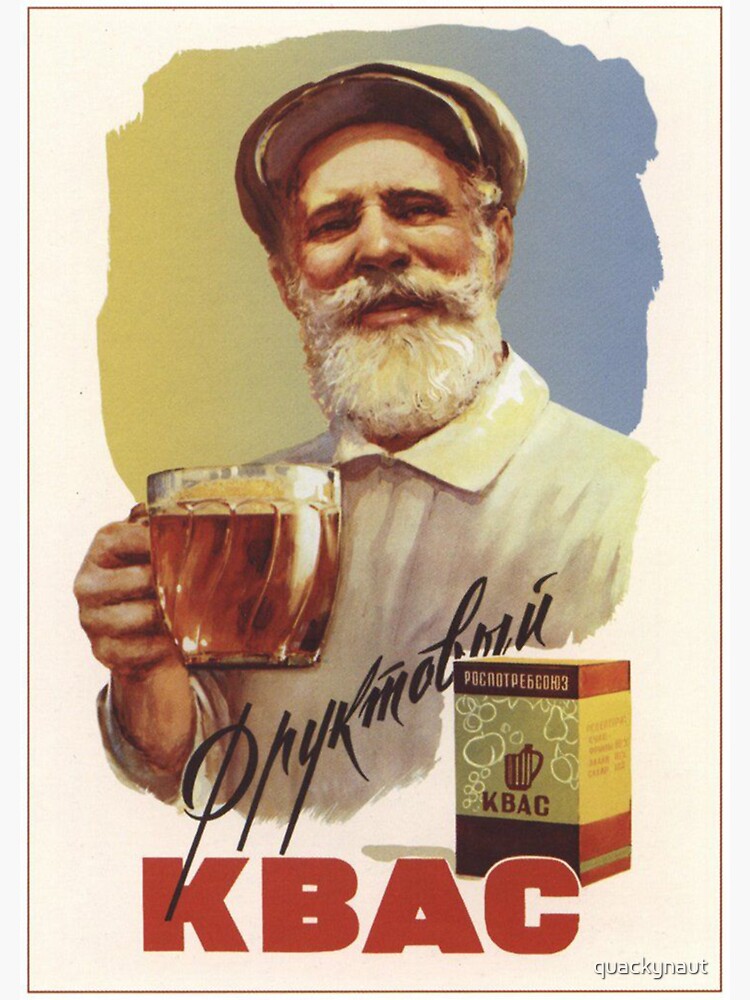The image features an advertisement in a foreign language, possibly Russian, for a beverage. The ad prominently displays an older man with a full white beard and mustache, reminiscent of Santa Claus, wearing a white collared shirt and a newsboy cap or beret-style hat. He is holding up an oversized glass cup filled with the beverage, which is larger than his fist. The name of the product, "KBAC," is written in large red letters on the packaging, which has a tan base color with red accents at the top and bottom. Surrounding the man are white outlines of various fruits, including pears, apples, grapes, cherries, and peaches. There is also a gradient splash of paint in the background that transitions from yellow to blue. Additional text appears on the ad, including something that looks like "Prykinobar" and another string of characters that seem non-English, adding to the foreign language context.